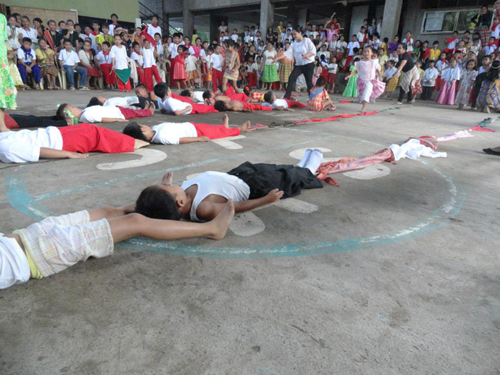In the image, a peculiar scene unfolds on a large cement floor that appears to be part of a sports court, suggested by visible lines possibly indicating a basketball court. In the foreground, several rows of children are lying down, extending from left to right with their bodies arranged head-to-foot. Starting from the left, one child's legs and bare feet enter the frame, with another child's head positioned near the first child's feet, creating a somewhat puzzling pattern. In each row, at the end of the last child's feet, there is a string of clothes and sheets tied together, extending for about 10 feet. This unusual arrangement is repeated in at least four visible rows. A person in a white shirt and black pants stands above them, apparently giving directions. Surrounding this scene, a multitude of people, predominantly children, form a crowded background that resembles a school environment, as indicated by the visible structure in the distant backdrop. The entire tableau hints at a demonstration or participative activity, though its exact purpose remains unclear.